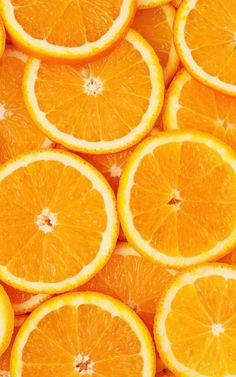This photograph captures a detailed, zoomed-in view of a rectangular array of thinly sliced, overlapping navel oranges. The slices, which lack any visible seeds, are meticulously arranged in stacks and rows, creating a layered pattern. Each orange slice is characterized by a vibrant, bright orange outer edge, a thicker white circumference, and a center made up of symmetrical orange triangles converging towards a white core. Despite slight variations, with some centers appearing partially disrupted, the overall impression is one of uniformity and fresh, bright citrus. The composition focuses solely on these orange slices, filling the entire frame and showcasing their intricate details and the interplay of layers from a top-down perspective.